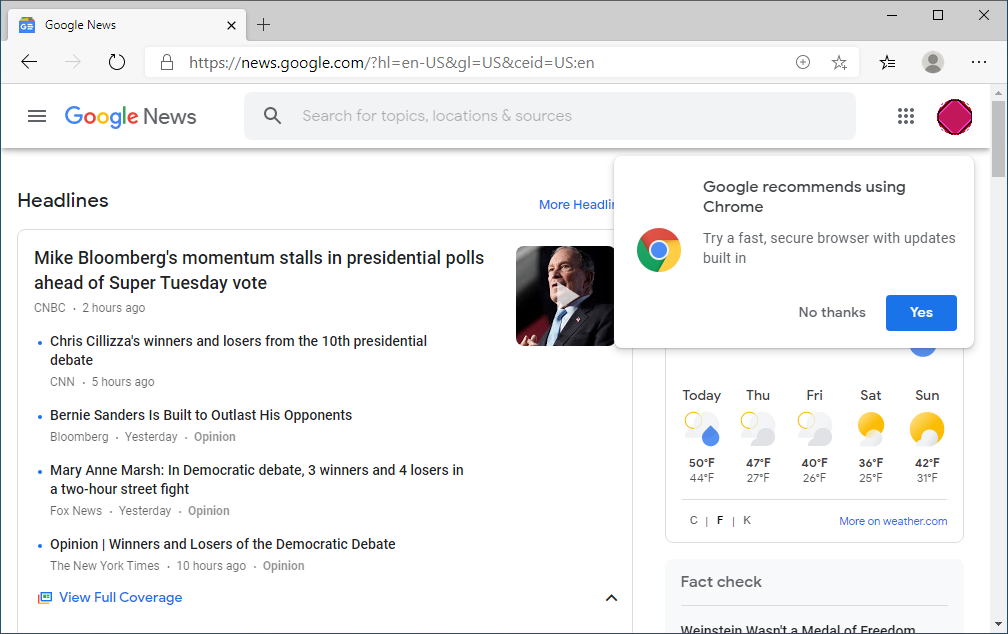A screenshot captures a Google News page displayed within a web browser. The browser window has a single tab open featuring the Google News landing page, identifiable by the "Google News" label on the left side. The URL bar reveals the typical structure of a Google News link. An overlay message from Google suggests using Chrome for a faster, more secure browsing experience, offering options to either decline or agree.

The main body of the page displays various news headlines. The top headline reads: "Mike Bloomberg's momentum stalls in presidential polls ahead of Super Tuesday vote" from CNBC, published two hours ago. Below it, a list of additional headlines includes:

- "Chris Cillizza's winners and losers from the 10th presidential debate," CNN, five hours ago.
- "Bernie Sanders is built to outlast his opponents," Bloomberg, yesterday (opinion piece).
- "Mary Ann Marsh: In Democratic debate, three winners and four losers in a two-hour street fight," Fox News, yesterday (opinion piece).
- "Opinion: Winners and losers of Democratic debate," New York Times, ten hours ago (opinion piece).

A "View full coverage" link provides further exploration options for these topics.

On the right side of the page, a weather forecast indicates current and upcoming weather conditions. Starting from today, which is Wednesday, the forecast extends through Thursday, Friday, Saturday, and Sunday, with low temperatures ranging from the 30s to the 50s, suggesting a springtime climate.

Beneath the weather section, a "fact check" section is visible, though specific details are not provided in the description.